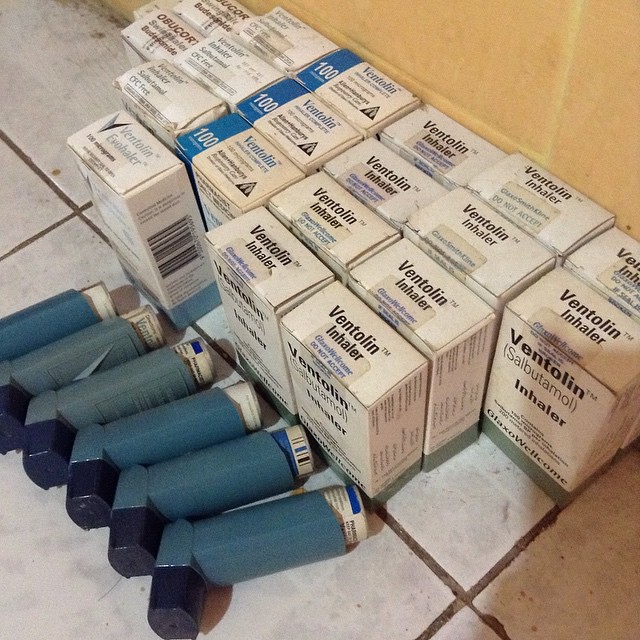The image showcases a dirty white tiled floor with a manila yellow back wall. In front of this wall are numerous medication inhalers, predominantly Ventolin inhalers, some in boxes while others are unboxed. Starting from the right, there are ten boxed Ventolin inhalers, grouped as two single boxes, followed by two sets of four boxes each, with a blue stripe indicating a dosage of 100. Adjacent to these, but without specific details, some additional unboxed Ventolin inhalers can be seen. Among the boxes, there are also a few inhaler boxes labeled OSC3 from Switzerland and two red and white Osocort inhalers. In the lower left-hand corner, six unboxed dark blue inhalers with navy blue caps are arranged, ready for use. The overall arrangement displays a somewhat chaotic assortment of inhalers against the backdrop of the tiled floor and wall.